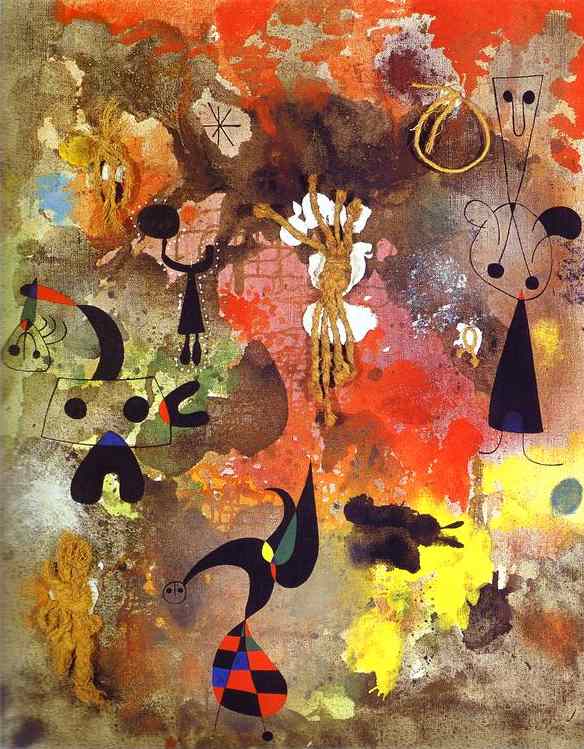The artwork is a whimsical and abstract mixed media piece characterized by a chaotic yet intriguing assembly of colors, shapes, and textures. The background is an energetic mix of orange, purple, yellow, brown, and black splotches, creating a vibrant and eclectic canvas. Layered upon this colorful base are a variety of simplistic, hand-drawn figures rendered in ink. These figures are abstract human-like forms, featuring geometric shapes such as triangles, circles, and rectangles for bodies, heads, and limbs. Many of the characters sport dot eyes and minimalist facial features, giving them a playful and surreal appearance.

On the upper right, there is a simplistic figure with a triangle body and a circle head, complete with dot eyes and ears. Adjacent to this figure is another with an upside-down triangular head and an oval body. In the middle, a distinctive character has a checkered pattern on its belly, resembling a whimsical creature with spider-like legs and a blob-like structure. The lower left corner features another brown figure with two legs.

The artwork is further embellished with physical elements, including brownish yarn and pieces of rope tied into various knots and glued onto different parts of the canvas, with notable placements in the upper right, middle, and lower left regions. These tactile additions extend the painting beyond mere visual stimuli, adding a layer of texture and dimensionality to the overall composition.

Altogether, the painting presents an eclectic mix of non-representational elements, geometric characters, and textural additions, embodying a sense of playful abstraction and imaginative expression.